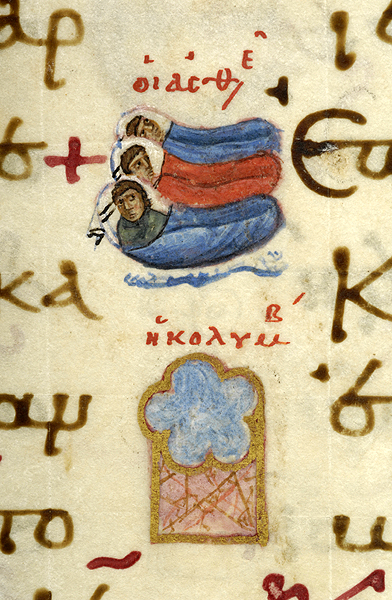The image appears to be a detailed illustration that likely comes from an old, possibly religious manuscript. The background is a yellowish-beige color, giving it an aged appearance. Surrounding the main illustration are writings in an unfamiliar language, which might be Russian or another language, written in brownish ink along the left and right edges.

Centrally featured are three men, each seemingly tucked into sleeping bags—the left and right ones are blue, and the middle one is red. These men are lying horizontally and staring in different directions, with their faces prominently shown. The illustration style resembles traditional Russian iconography.

Below the three men is a decorative element that looks like a blue, gold-accented, star-shaped floral design, reminiscent of stained glass. Underneath this design, there is a pink rectangular area filled with red, scribble-like markings that add to the image's intricate detail. This entire scene looks like something you might find displayed in a museum as part of an ancient, religious artifact collection.